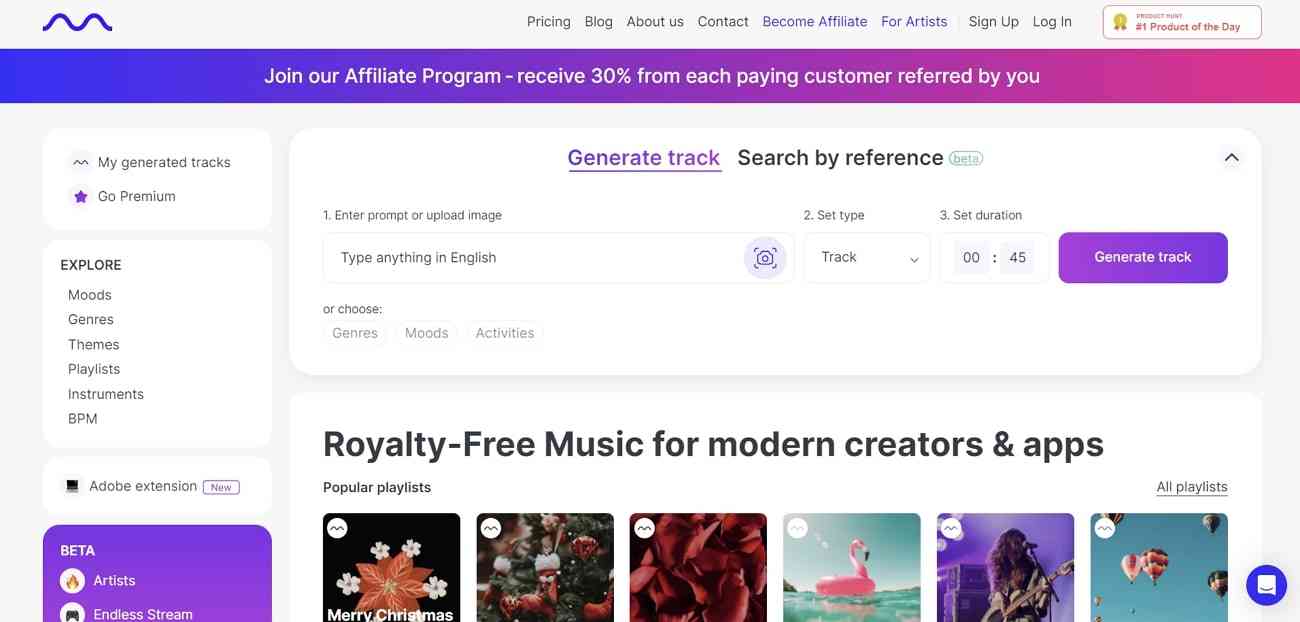**Detailed Caption:**

This image is a detailed screenshot from a music generation website, showcasing a variety of user options and navigation features.

At the very top of the page, there is a horizontal menu bar offering links to key sections such as Pricing, Blog, About Us, Contact, Become an Affiliate, For Artists, Sign Up, and Login. 

Directly below this menu, a prominent banner invites users to "Join Our Affiliate Program," highlighting an offer to receive 30% from each paying customer referred by the user.

On the left-hand side, a vertical navigation panel presents additional links categorized as My Generated Tracks, Go Premium, Explore, Moods, Genres, Themes, Playlists, Instruments, APM, and Adobe Extension.

In the center of the page, the website offers a variety of interactive options designed to assist with music creation. These options include "Generate Track," "Search by Reference," "Input or Upload Image," and "Type Anything in English." Users can also set specific parameters such as track type, duration (example given is 0 minutes and 45 seconds), and choose from genres, moods, and activities.

At the bottom of the central section, the page describes its service as offering "Royalty-Free Music for Modern Creators and Apps" and features a "Popular Playlist."

The overall design of the website is encapsulated within a rectangular frame.